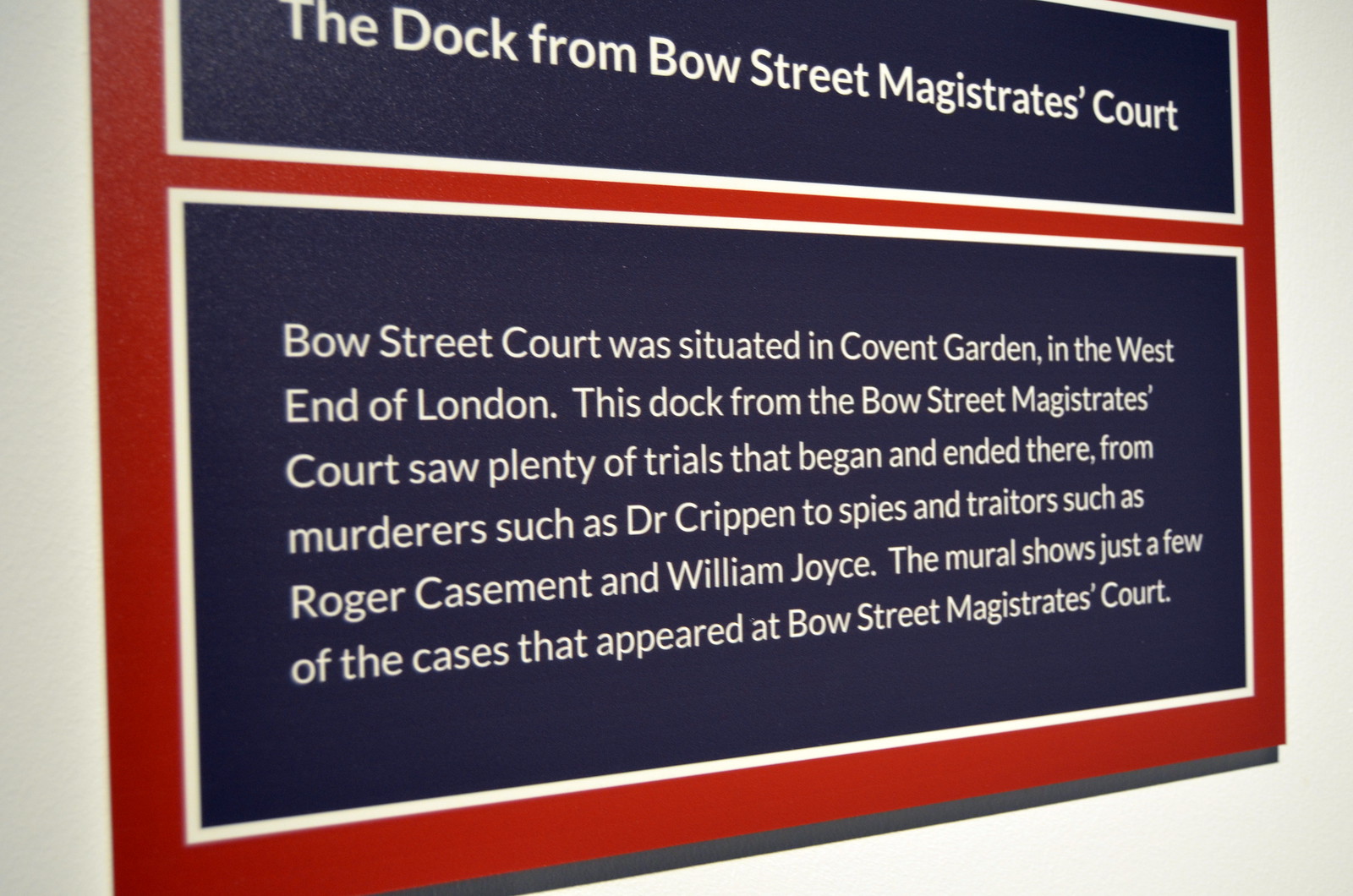This image captures a color photograph of an informational plaque mounted on a white wall. The plaque features a red background with two prominent horizontal blue blocks outlined in white. In the top blue block, white letters read, "The Dock from Bow Street Magistrates Court." Below this, a larger blue box contains additional text in white: "Bow Street Court was situated in Covent Garden in the West End of London. This dock from the Bow Street Magistrates Court saw plenty of trials that began and ended there, from murderers such as Dr. Crippen to spies and traitors such as Roger Casement and William Joyce. The mural shows just a few of the cases that appeared at the Bow Street Magistrates Court." The photograph is taken at a slight angle, causing the left side of the plaque to appear larger than the right due to the perspective. The plaque is the focal point of the image, providing historical context with a clean, professional presentation.